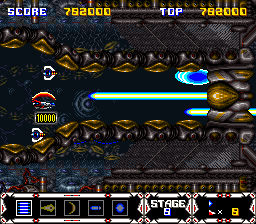The image depicts a classic, retro video game screen characterized by pixelated graphics. The main focus is a blue beam emerging from a brown object, set against a backdrop filled with brown and gray structures that resemble the intricate lining of a creature's cavity. To the left, a red spherical object displays the number "10,000" beneath it, signifying either points or an in-game item. Surrounding this red sphere are small, finned blue spaceships. The HUD at the top of the screen shows the player's score as "752,000," which is also their top score, indicating that they have achieved a new personal best. The current game stage is labeled as "Stage 5," suggesting that the player is progressing towards Stage 6 out of a total of 99 stages, finally nearing a significant milestone.